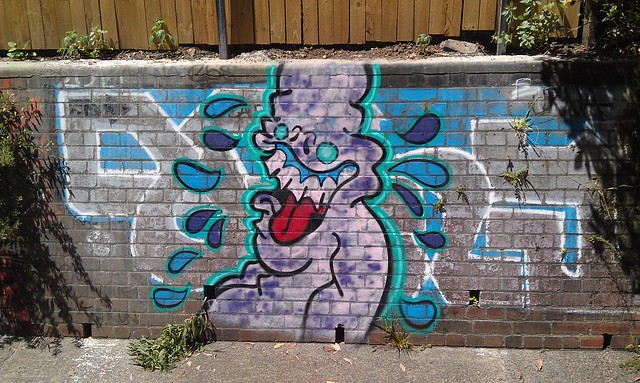The image depicts a vivid piece of graffiti adorning a concrete retaining wall topped with a wooden structure. The central figure in the artwork is a grotesquely charming, lumpy, purple character with a large head, laughing with its mouth wide open, revealing a prominent red tongue and exposed teeth. The character has expressive blue eyes, matching the neon teal outline around it, and is highlighted by light and dark blue droplets that could symbolize sweat or tears of joy. The scene is set outdoors, with a concrete sidewalk and green weeds sprouting through the cracks in front of the wall, providing a gritty urban backdrop to the playful and stylized street art.